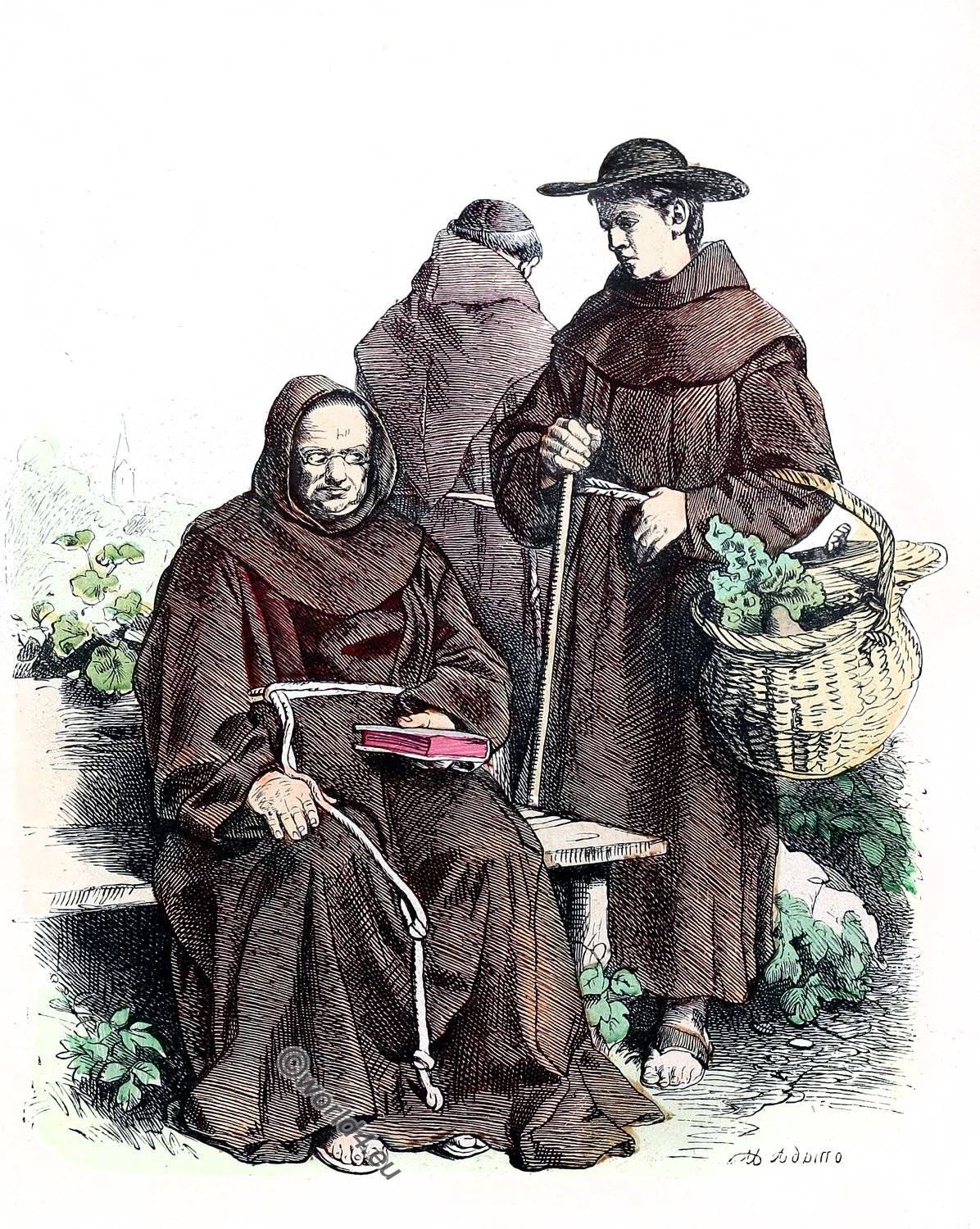The illustration depicts a serene outdoor scene featuring three figures dressed in long, brown robes tied with white ropes at the waist, set against a white background. A central, older man sits on a white bench, holding a book that likely represents a religious text such as the Psalms or the Bible. His expression is one of surprise as he gazes at a younger boy beside him, who is clad in a black hat and holds a wicker basket filled with vegetables. Positioned slightly in the background and turned away is a third figure, also garbed in a similar robe, contributing to a sense of contemplation. Around them, the vegetation of a lush garden with small plants and green shrubs adds to the tranquil and spiritual atmosphere. The image, suggestive of a serious conversation, feels set within a religious or monastic context. Details such as the artist's signature in the bottom right corner and a watermark labeled "4.EU" at the bottom center corroborate its artistic authenticity.